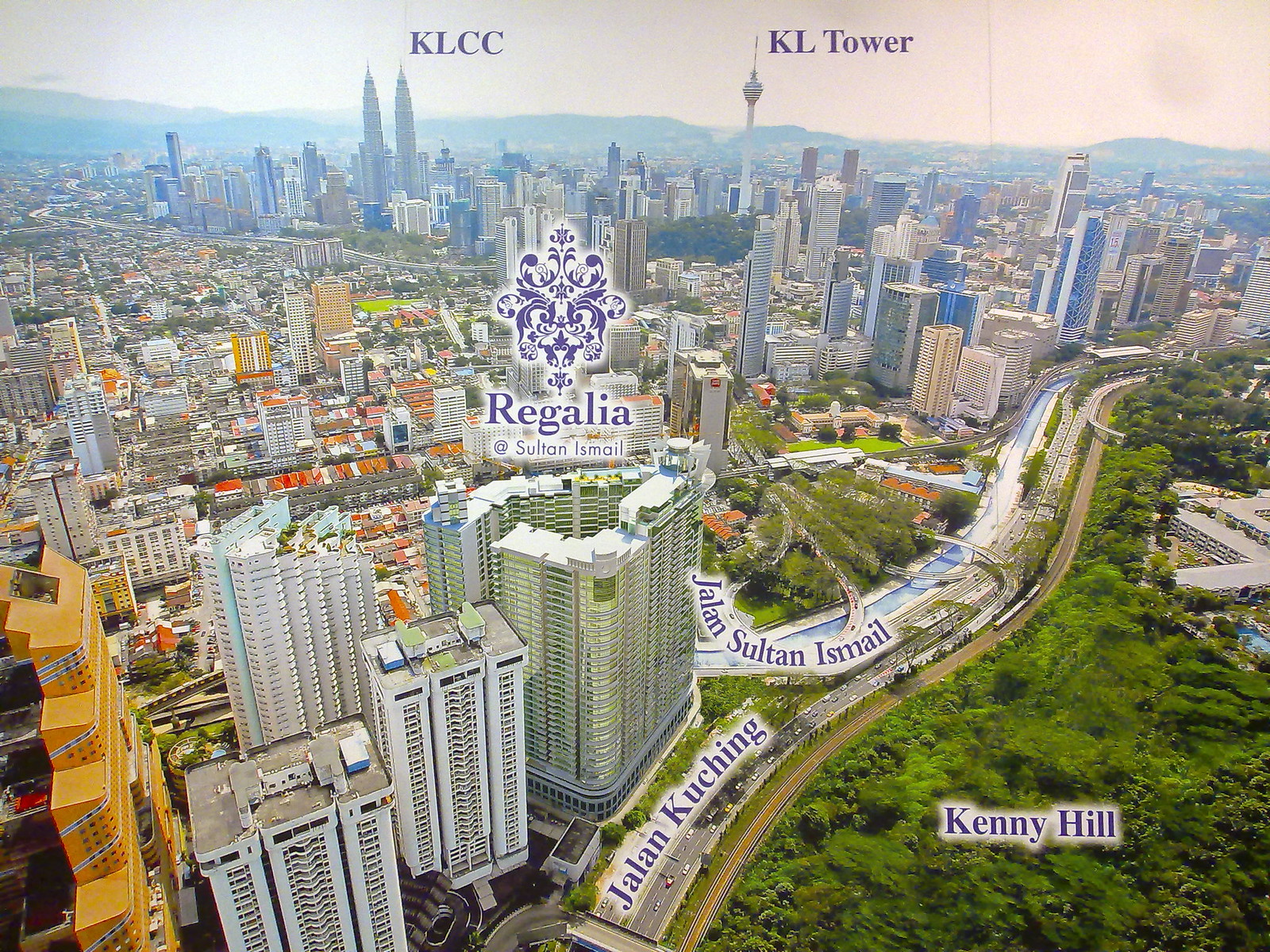This is an aerial photograph of an urban area, prominently detailing several labeled locations and landmarks. The photograph, taken from a high angle, captures a bustling cityscape with multiple tall buildings and a comprehensive view of the skyline. In the background, you can see numerous multi-story urban buildings and a range of mountains that add depth to the scene. Towards the top of the photo, the iconic twin towers labeled KLCC and the needle-like structure labeled KL Tower demark significant points of interest in the city. 

At the center, slightly off-center is a notable high-rise building that is likely a hotel, labeled "Regalia Sultan Ismail" in a blue design with a logo adjacent to it. The area around this building is densely populated with other high-rises. Below this, several main roads intersect the urban landscape, with key roads labeled in blue lettering on a white background; these include Jalan Kuching and the rounded freeway-like Jalan Sultan Ismail. 

In the lower right-hand corner, a green, forested area marked "Kenny Hill" provides a contrast to the urban expanse, with both a road and a river running along its edge. Collectively, the details indicate that the photograph likely depicts a cityscape in Malaysia, showcasing the vibrant mix of natural and urban features in the region.